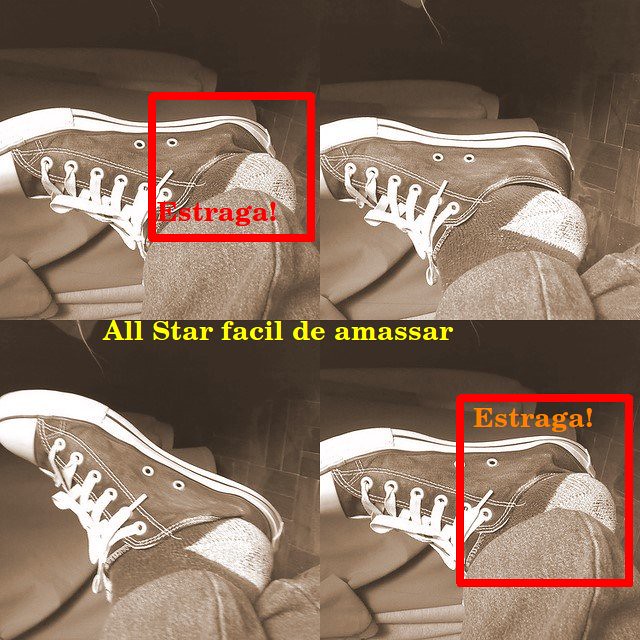The image is divided into four quadrants, arranged in a two-by-two grid, each showcasing a slightly different angle of a person's partially worn sneaker. The photos exhibit a brown hue, giving them a sepia-toned aesthetic. In the upper left quadrant, the sneaker features a white toe cap, white sidewalls, and white laces, with a denim-like texture. The person's foot, half in the shoe, is adorned with black and white socks, and there's a red square with the word "ESTRAGA!" overlaying the photo. Moving to the upper right quadrant, the scene is almost identical, highlighting more of the floor, which appears to be made of brick, and a bit more of the person's jeans. The lower left quadrant mirrors the upper right one with no significant differences. In the lower right quadrant, akin to the upper left, there's a shoe similarly positioned, with a bigger red square containing "ESTRAGA!" in orange text. Across the middle of the bottom two photos runs the phrase "All Star FACIL DE AMASSAR" in yellow letters, hinting at it being an advertisement. Overall, the image forms a collage focused on the sneaker and its varying positions.